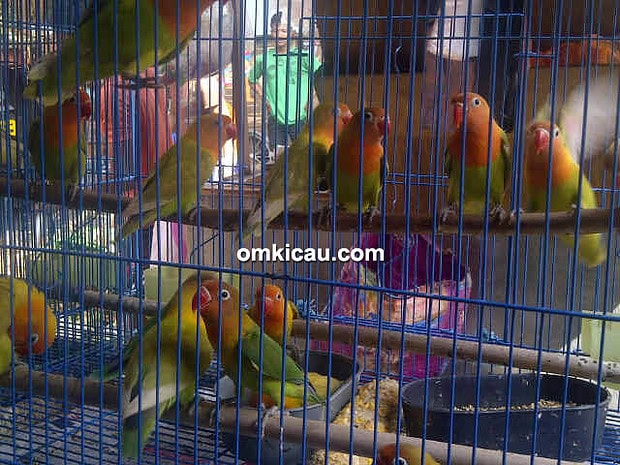The photograph captures a rectangular birdcage with distinctive blue bars, both vertical and horizontal, filled with numerous identical birds. Each bird features a vivid blue feathered body complemented by an orange or yellow head and neck, with curved orange beaks and small black eyes. Their gray feet and legs grip onto smooth brown dowels arranged inside the cage. Approximately ten birds are scattered throughout the cage, perched in varying positions on these dowels, with some facing forward and others turned away. 

At the bottom of the cage, a blue grate covers yellow straw or plant material. Placed centrally on this grate are two blue trowels—one containing seeds and the other holding a yellow substance. Positioned between the trowels lies a partially eaten corn cob, most of its kernels removed. Additionally, there are people visible behind the cage, possibly indicating it is located in a pet store environment. The cage also prominently features the text "omkicau.com" in white lowercase letters, centered at the top. The colorful scene incorporates a variety of hues, including red, orange, green, brown, dark blue, light blue, white, and black.